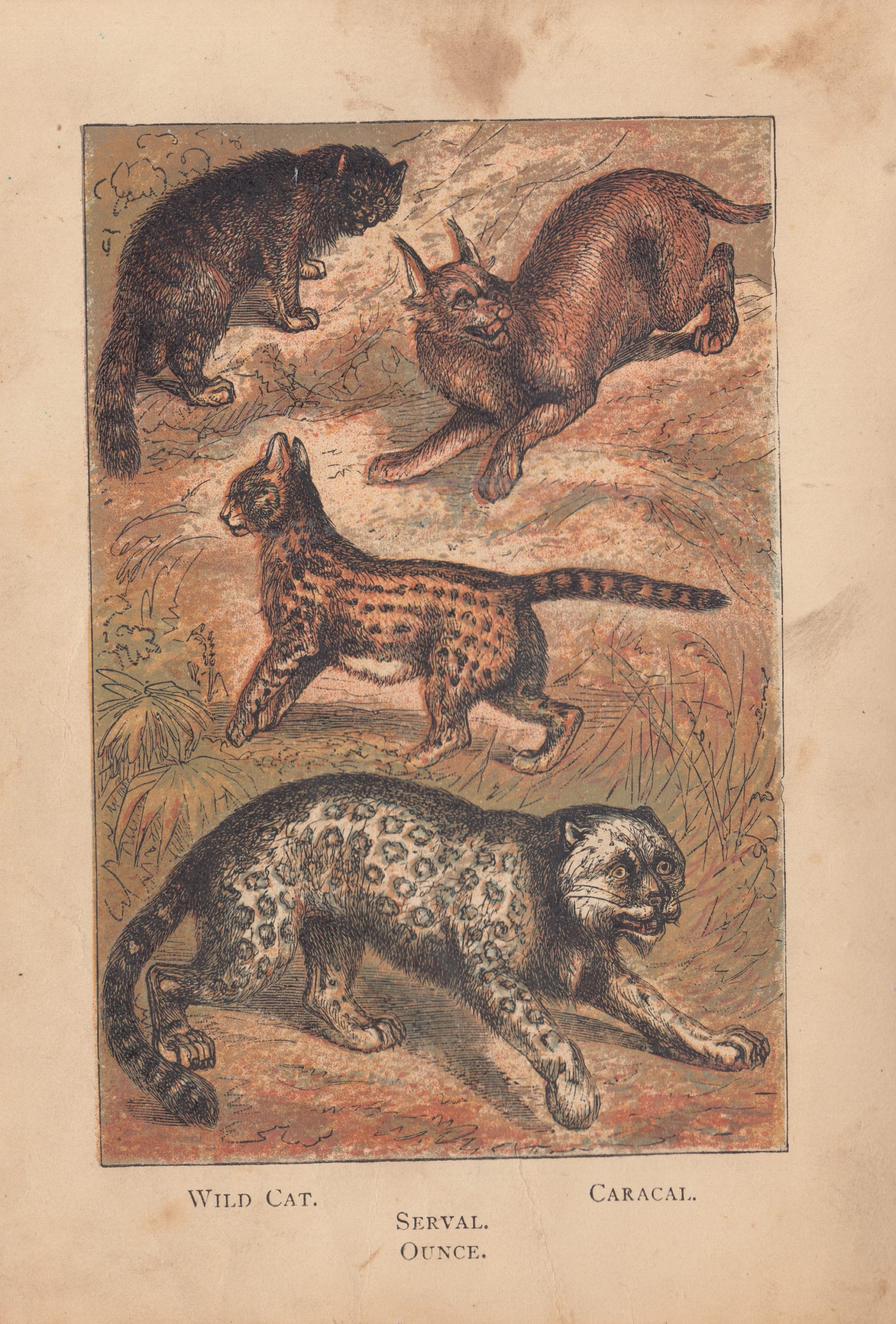This detailed illustration appears on aged, light brown paper that shows noticeable wear and darker brown spots around the edges. It depicts a vertical rectangle sketch colored with ink and shows four different animals arranged one above the other. At the bottom, facing right, is a large leopard, characterized by its goldish-brown color and distinct black-bordered spots. Above it is a baby tiger or cub, orange-colored with brown spots, facing left. At the top left sits a grayish-black house cat, while the top right features an animal with long, pointy ears, initially mistaken for having horns but likely a brownish-orange dog. The paper is visibly dirty, enhancing its vintage appearance. The bottom of the illustration has text identifying the animals from left to right: wildcat, serval, ounce, and caracal.